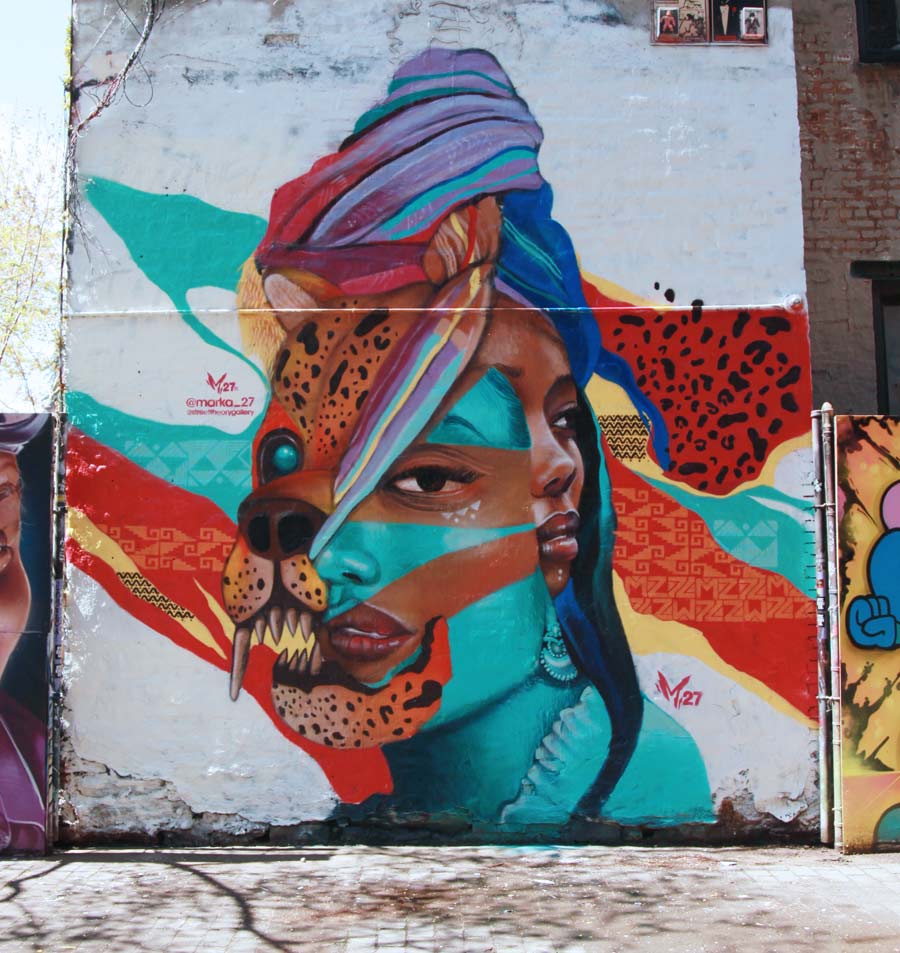This image is a detailed color photograph of an outdoor wall mural painted on a red brick building. The mural, set against a distressed white background, features an intricate and vivid portrayal blending human and animal forms. Dominating the composition is a central image of a shape-shifting entity with a striking half-leopard, half-human face. The leopard side is adorned with brown fur, a blue eye, and sharp fangs, while the human half depicts an African American woman with brown skin, dark red lips, and a partially blue-painted face. She has three white triangles beneath her eye and brown eyes. Nearby, another woman's partial profile with a brown complexion is visible, gazing rightward. She wears a vibrant, turban-style head wrap in shades of blue. Surrounding the figures, abstract shapes and stripes of red with black leopard spots, aqua, yellow, red with orange triangles, and more aqua hues add dynamic energy to the scene. The mural extends to the left portion of the wall, featuring additional smaller graffiti elements and colorful abstract forms. Trees behind the building cast shadows on the cobblestone or brick-paved sidewalk, adding depth and context to the vibrant urban setting. There is also tiny text within the mural, although it is too small to decipher.